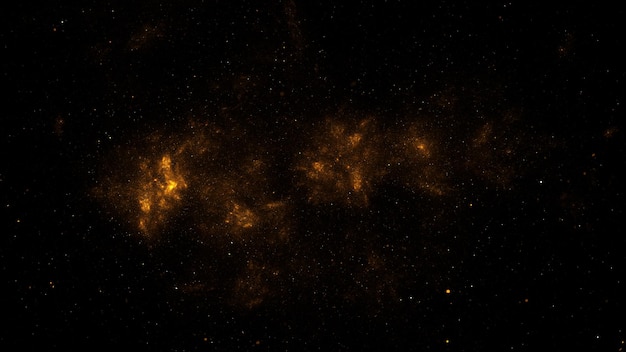The image depicts a captivating view of outer space, characterized by a predominantly dark, almost entirely black night sky. Scattered throughout the expanse are numerous glistening white stars, along with some that have hints of amber. At the center of this cosmic scene is a swirling nebula with a dreamy, ethereal quality. The nebula glows with vibrant hues of orange, yellow, and gold, creating an impression of illuminated atmospheric gas or clouds. This central formation appears almost cloud-like in structure, with darker, bronze-brown edges dissolving into the inky blackness. The vividly bright amber and darker tones around it evoke a sense of wonder and the mysterious beauty of galactic phenomena. The overall composition is one of minimalism, dominated by the vast, empty darkness of space punctuated by the few bright stars and the luminous nebula at its heart.